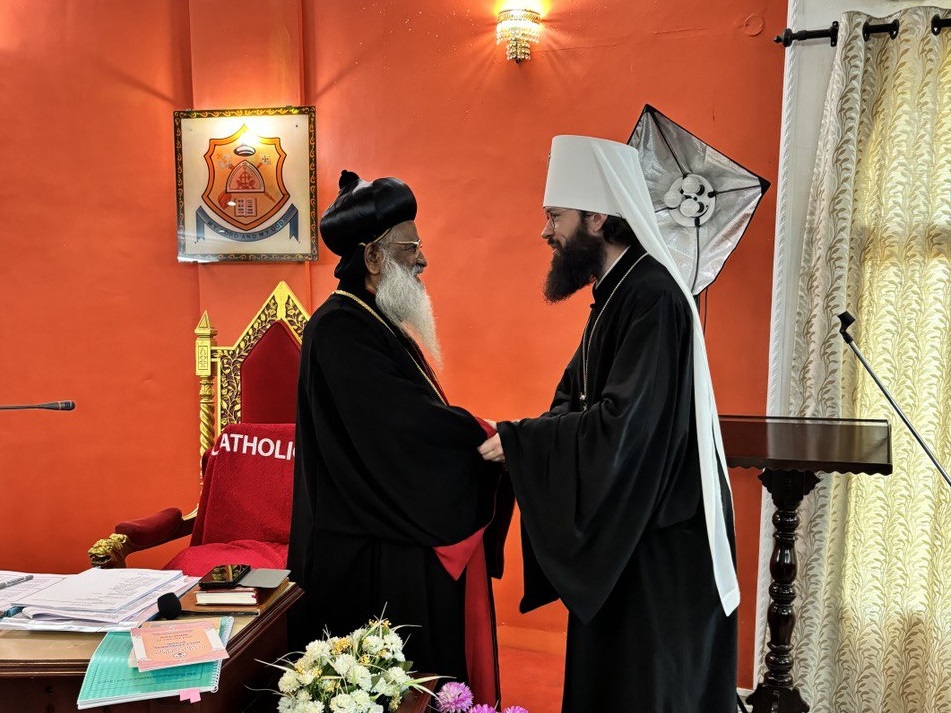In a warmly lit room with orange walls and off-white curtains, a detailed scene unfolds. A yellow light fixture casts a gentle glow over a golden and red throne, which sits beside a cluttered desk adorned with papers in blue, white, black, and pink. Scattered around the desk are vibrant white, yellow, and pink flowers, accentuated by the presence of a black wooden pulpit. 

At the heart of the image, two men warmly clasp hands, their faces lit up with mutual smiles. Both wear glasses and are dressed in black robes. On the left stands a light-skinned man with a black beard, wearing a distinctive white cylindrical hat, reminiscent of an upside-down popcorn container, with a white scarf cascading from it. He appears to be a Roman Catholic priest. Opposite him, on the right, is a brown-skinned man with a gray-white beard extending halfway down his chest, wearing a pointed black hat adorned with gold stripes around the neck of his robe, identifying him as a Muslim religious leader. Both figures stand in profile, highlighting their harmonious encounter. Behind them, a red fabric inscribed with the word "Catholic" in white, and a picture with an indistinct symbol, creates a colorful backdrop to this moment of interfaith camaraderie.